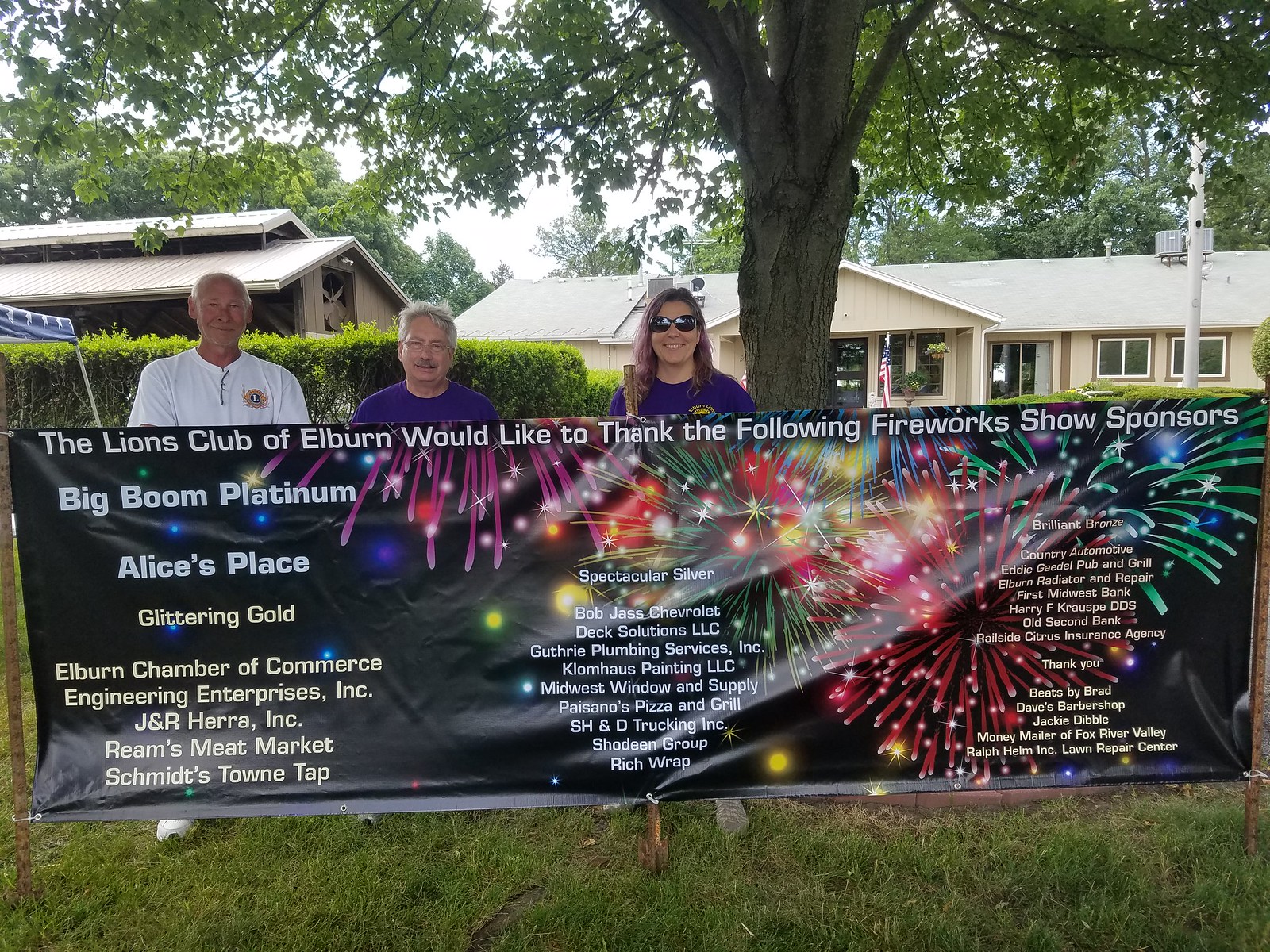In this vibrant full-color outdoor photograph taken during the daytime, three individuals—a man in a white crew neck shirt, a man in a purple t-shirt, and a woman in a purple t-shirt with sunglasses—stand on a grassy area under a tree. They are in front of some bushes and two single-story buildings—one with an American flag and likely to be either a house or a depot given the railroad crossing sign visible nearby. Across the entire width of the photo, the three are holding a large banner adorned with colorful fireworks in shades of purple, orange, green, red, yellow, white, and blue. The banner, which has text layered over the fireworks display, reads: "The Lions Club of Elburn would like to thank the following fireworks show sponsors." Listed prominently are sponsors such as Big Boom Platinum, Alice's Place, Glittering Gold, Elburn Chamber of Commerce, and many others in varied font sizes due to the extent of the list. This image serves as a thank-you post-event for the town’s Fourth of July fireworks, recognizing the significant community support.